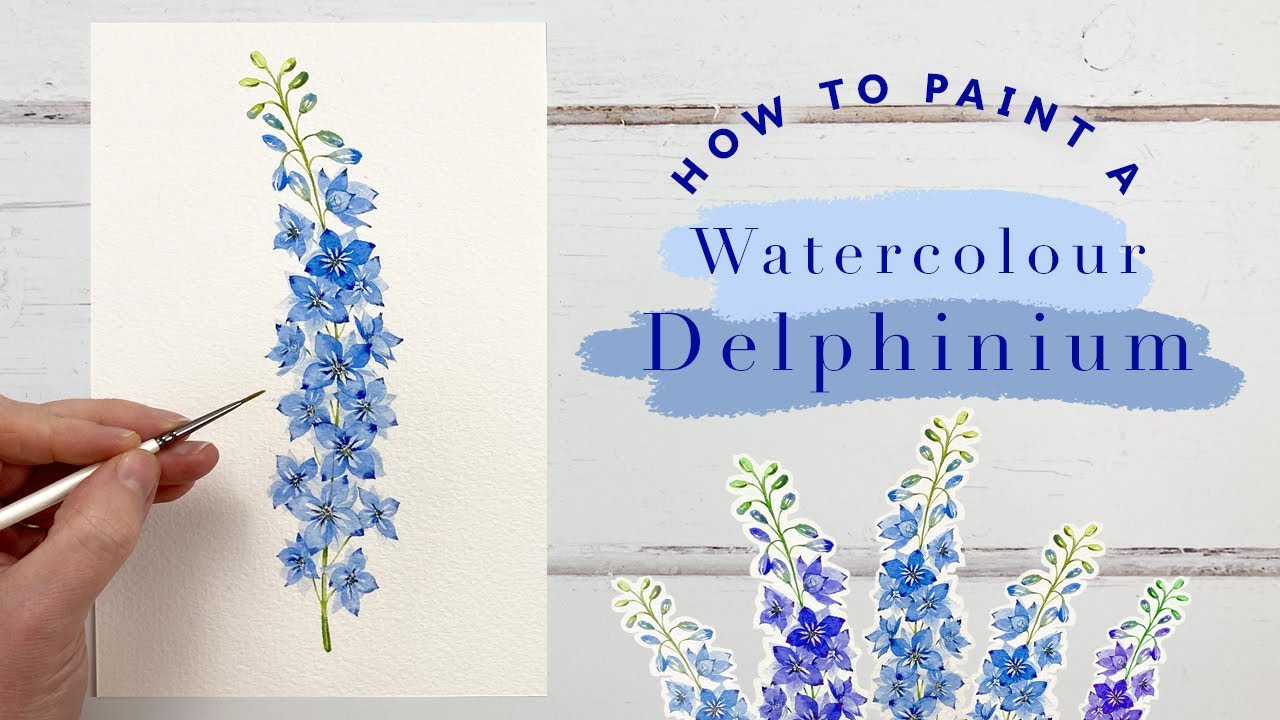The image portrays an artist's detailed watercolor painting tutorial. On the left side, a white piece of watercolor paper features a delicate painting of a delphinium plant. The plant is characterized by long stems, vibrant blue flowers near the base, and green buds at the top. A hand, presumably of the artist, is visible holding a thin, white and silver paintbrush, poised over the painting. 

On the right side of the image, three lines of text are prominently displayed. The phrase "how to paint a" is written in an arch, instructing viewers on the topic. The words "watercolour delphinium" are highlighted, with "watercolour" printed in blue over a baby blue swatch and "delphinium" in a muted blue color. Below the text, there are illustrations of various delphinium flowers in different shades of blue and purple, serving as examples or inspiration. The background of the image appears to be a white wooden table, suggesting a clean, organized workspace, typical for an instructional video or a YouTube tutorial.